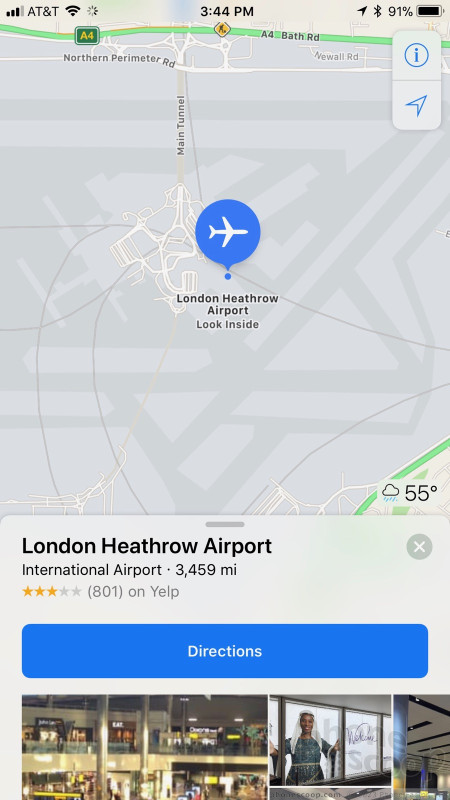This screenshot captures a range of detailed information from a person's cell phone. In the top-left corner, it reveals that the user has three bars of network coverage under the AT&T carrier, is connected to Wi-Fi, with the current time being 3:44 p.m. and the battery level at 91%. 

Dominating the center of the image is a map, predominantly gray and white, with a prominent blue circle at its center featuring a white airplane icon flying to the right, indicating London Heathrow Airport. Beneath this icon, there is a label that reads "London Heathrow Airport. Look inside." 

In the bottom-right corner of the map, the weather is noted as 55 degrees Fahrenheit with a rain cloud icon showing precipitation. 

Below the map, the text "London Heathrow Airport. International Airport, 3,459 miles" is displayed, followed by a rating showing three out of five stars based on 801 Yelp reviews. 

A long blue rectangle with the word "Directions" in white lettering is prominently positioned in the center. Directly underneath, partially visible photos showcase interior shots of the airport, including shopping areas and various signage. 

The screenshot is portrait-oriented and notably does not feature any animals.